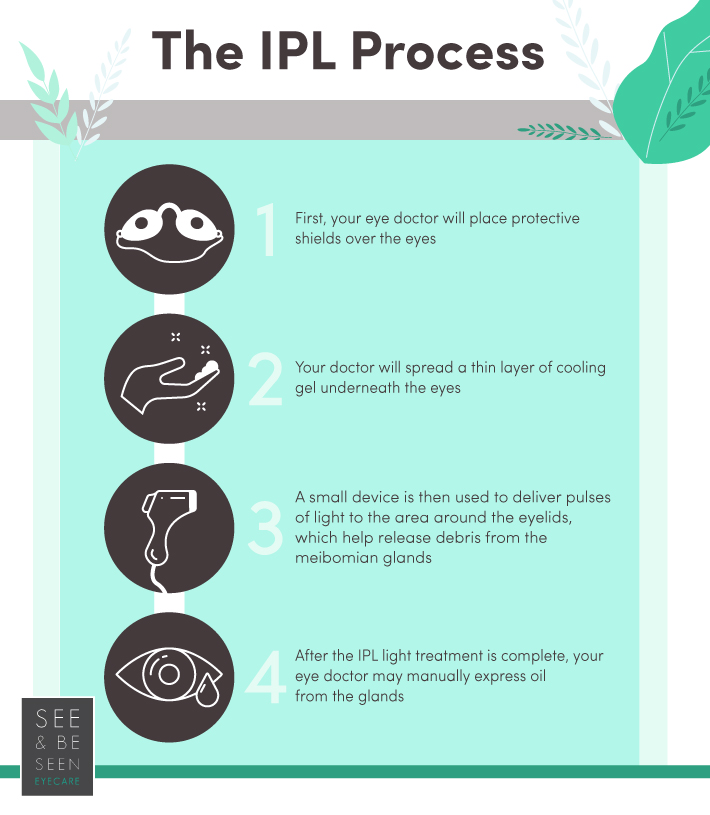The informational poster titled "The IPL Process" is displayed prominently at the top in dark brown or black font. Set against a very light green background, the poster is artistically framed with green leaves painted or drawn along the top and sides. It outlines four key steps of the IPL treatment using four dark brown numbered circles, each containing white text.

1. **Protective Shields**: An image shows eye protective shields, indicating that first, your eye doctor will place protective shields over your eyes.
2. **Cooling Gel Application**: The next step is depicted by a hand with sparkling gel, illustrating that your doctor will spread a thin layer of cooling gel underneath your eyes.
3. **Light Pulse Delivery**: A small device resembling a hair blow dryer is shown, used by the doctor to deliver pulses of light around the eyelids, which helps release debris from the meibomian glands.
4. **Oil Expression**: Lastly, an illustration of an eye with a tear drop indicates that, after the IPL light treatment, your eye doctor may manually express oil from the glands.

The poster concludes with a black sign framed with a green line at the bottom left, stating "See and Be Seen Eye Care" in white lettering.